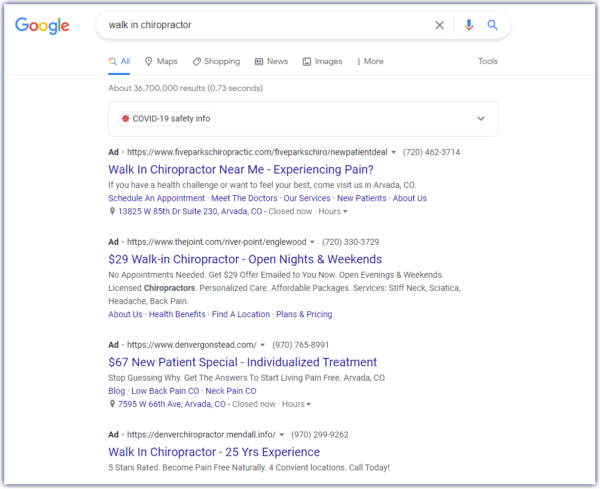A Google search query for "walk-in chiropractor" displays four prominent ad results at the top of the page, along with an expandable section for COVID-19 safety information. The highlighted results include:

1. **Five Parks Chiropractic**: An ad suggesting a solution for those experiencing pain with the search term "walk-in chiropractor near me."
2. **The Joint Chiropractic**: An ad promoting their walk-in services available during nights and weekends, featuring a $67 special for new patients.
3. **Denver Gonstead Chiropractic**: An ad emphasizing individualized treatment plans.
4. **Mendal Chiropractic**: An ad spotlighting their 25 years of experience.

The page follows the typical Google search layout with a clean, white background, blue hyperlinks, and black text. Additional search options for maps and news are available, along with phone numbers included at the end of each URL.